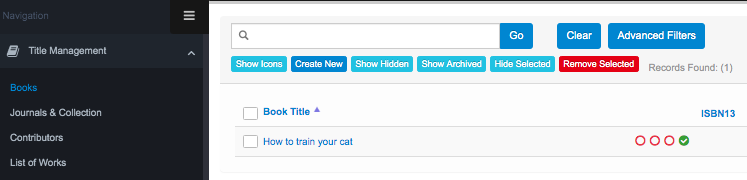Here is a cleaned-up and detailed descriptive caption for the image:

---

The screenshot depicts an interface of a media management application that could be on a desktop, laptop, tablet, or smartphone. The left-hand side features a dark blue navigation panel labeled "Navigation" at the top with three white horizontal lines indicating a settings menu. Adjacent to the navigation panel, the new section appears in a lighter blue shade, resembling a digital magazine or book interface. This section is titled "Title Management" in white text, accompanied by an upward arrow.

Below "Title Management," there are several hyperlinks in blue text, including "Books," "Journals," "Collection," "Contributions," and "Lists of Works." 

On the extreme right, there's a dark gray rectangular section containing a search bar. The search bar features a black magnifying glass icon on the left and a small dark blue button labeled "Go" on the right. To the right of the search bar, there are two dark blue buttons labeled "Clear" and "Advanced Filters," respectively. 

Within the new section are several cascading action buttons: the first one is cyan blue and says "Show Loans" in white text, followed by a dark blue button labeled "Create New." Next, there's another cyan button labeled "Show Hidden," then a dark blue "Show Archived" button, and another dark blue "Hide Selected" button. Finally, a red button with white text reads "Remove Selected."

Further down, it states "Records Found: 1" in gray parenthesis. Beside this, a blue-text hyperlink reads "Book Title" with an up arrow for sorting, and next to it, "ISBN 13" is displayed. On a new line, there is an unchecked square box next to a hyperlinked blue text reading "How to Train Your Cat." To the right are four circles indicating status—three are red, and the last one is green with a white check mark.